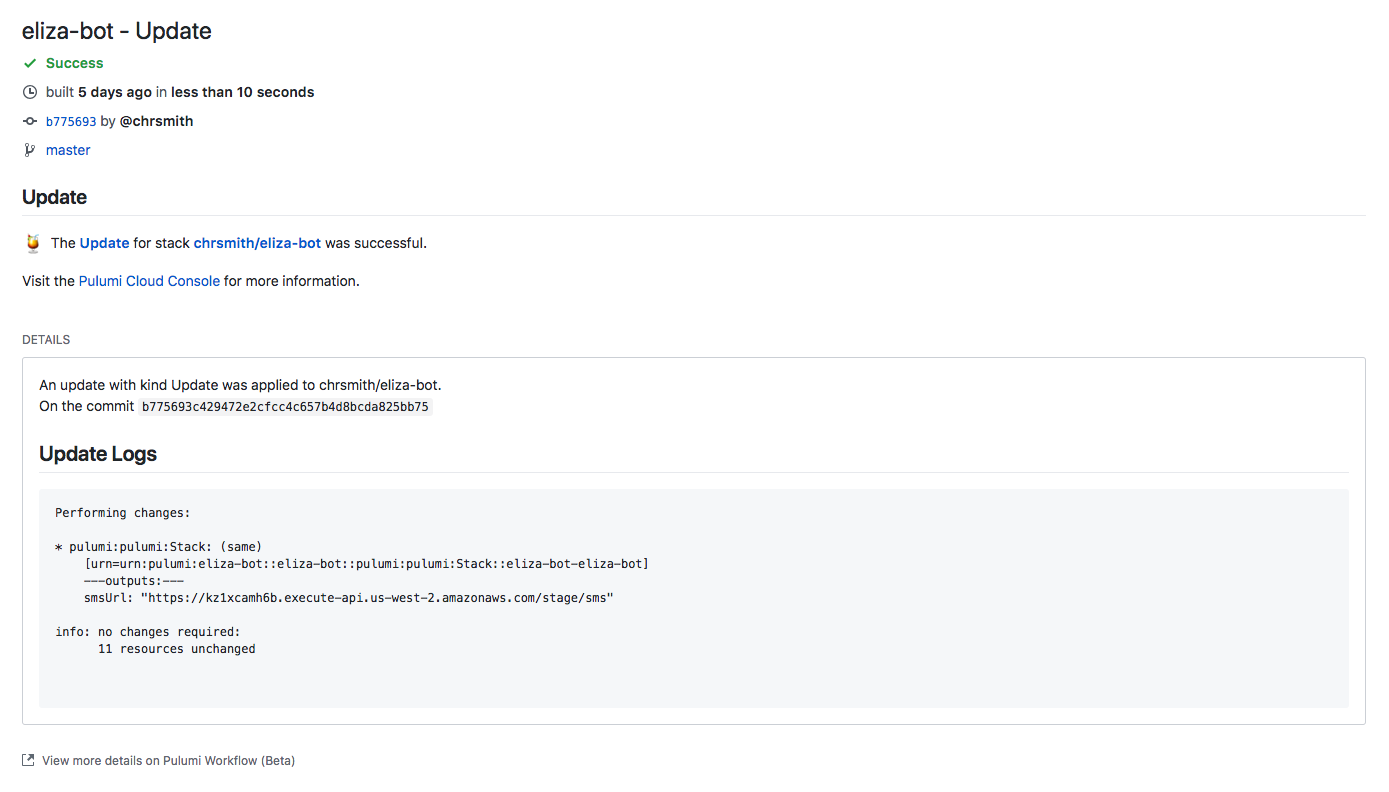The image depicts a web page with a clean, white background. In the upper left-hand corner, black text reads "ELIZA-BOT-UPDATE." Directly underneath, the word "SUCCESS" appears in light gray text, accompanied by a gray checkmark icon to its left. Below this, another line reads, "BUILT FIVE DAYS AGO IN LESS THAN 10 SECONDS," also in light gray text.

Proceeding further down, bright blue text displays the code "B775693." The subsequent line states, "BUY AT CHRIS SMITH, CHRSMITH," in black text. Following this, "MASTER" is written in blue text, and below that, the word "UPDATE" is in black text with a capital 'U.' A thin, pale gray horizontal line separates these sections.

The next portion of text states, "THE UPDATE FOR STACK CHRIS SMITH/ELIZA-BOT WAS SUCCESSFUL," in black text followed by, "VISIT THE PALOOMI CLOUD CONSOLE FOR MORE INFORMATION," with "Paloomi Cloud Console" highlighted in bright blue text.

At the bottom, there is a horizontal rectangular box outlined with a thin, light gray border. Above this box, "DETAILS" is written in all capital letters. Inside the box, the text reads, "AN UPDATE WITH KIND UPDATE WAS APPLIED TO CHRIS SMITH/ELIZA-BOT. Next line on the commit," followed by a long sequence of numbers and letters, highlighted in light gray.